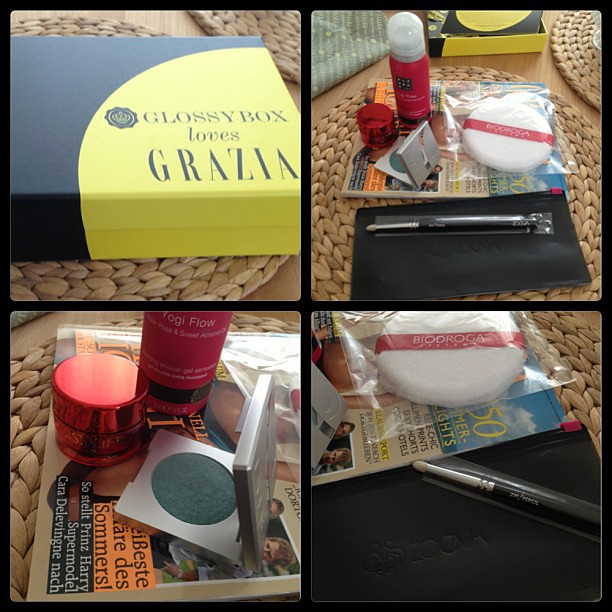The image consists of four sections, each showcasing various items atop a table. Centered around a glossy black box adorned with a yellow one-third circle and the text "Glossybox loves Grazia" in the top left corner, the scene depicts an unboxing of makeup and hygiene products, likely presented by an influencer. Spread out within these sections are diverse makeup goods — a small-headed makeup brush, white facial cleaning pads with a distinctive red stripe, a fine-grain black wallet, and a set of hygiene items labeled "Yogi Flow." Additionally, there are close-up shots of makeup palettes, presumed to contain blush or rouge, and other cosmetic implements, all placed on top of magazines. The arrangement and repetitive highlighting of makeup items against a wicker doily backdrop creates a detailed and engaging showcase for viewers.